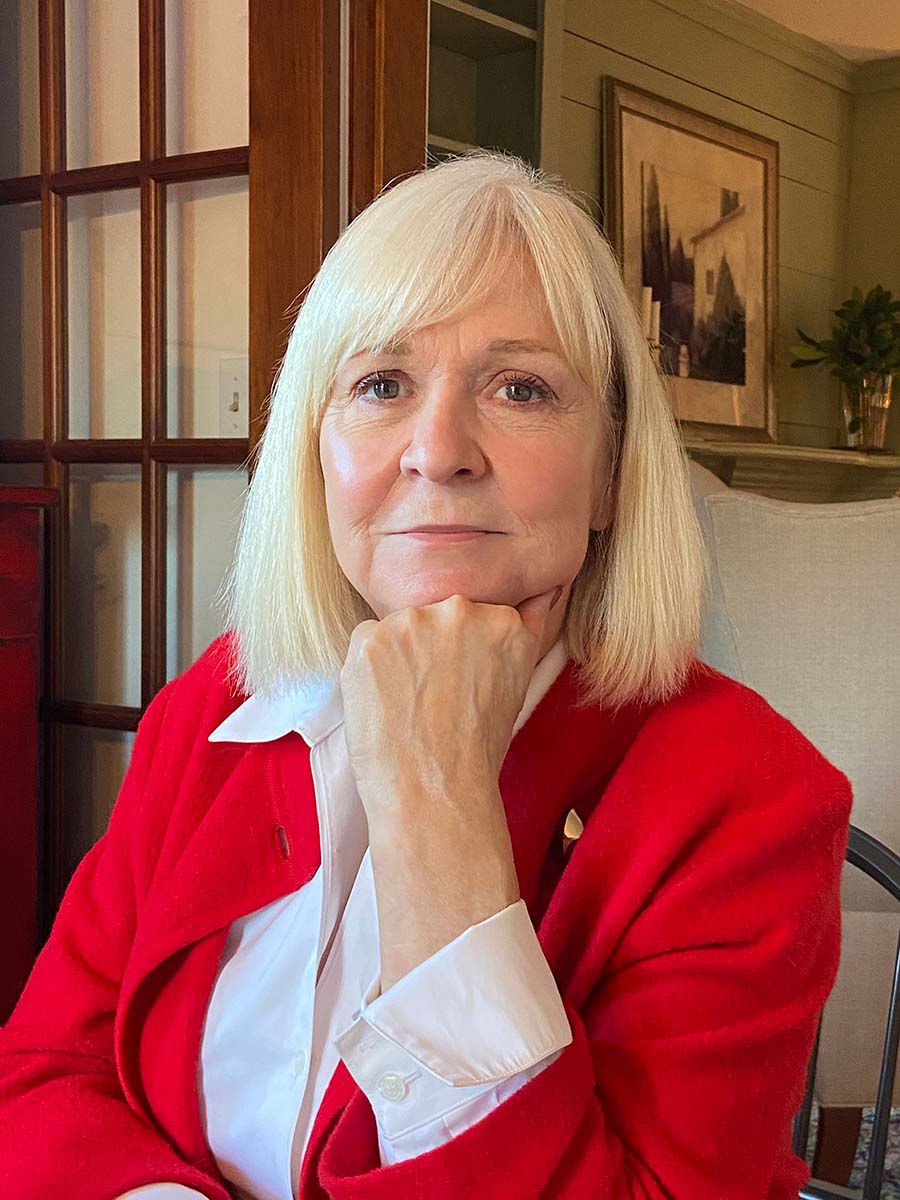This detailed portrait captures a woman in her 60s with platinum white hair, green eyes, and a very pale complexion, highlighting the marks of age including wrinkles under her eyes. She is seated on a black frame chair, posing thoughtfully with her head resting on her fist. The woman is elegantly dressed in a bright red overcoat that's unbuttoned, revealing a collared white shirt underneath, whose cuffs and collar overlap the thick red jacket. The setting is an interior room adorned with various elements—a painting of a house and trees hangs on an olive-colored wall, accompanied by a couch, a wooden door with window breaks, a green cabinet or entertainment center, a house plant, and a candle. The overall atmosphere exudes a warm, homely feel.